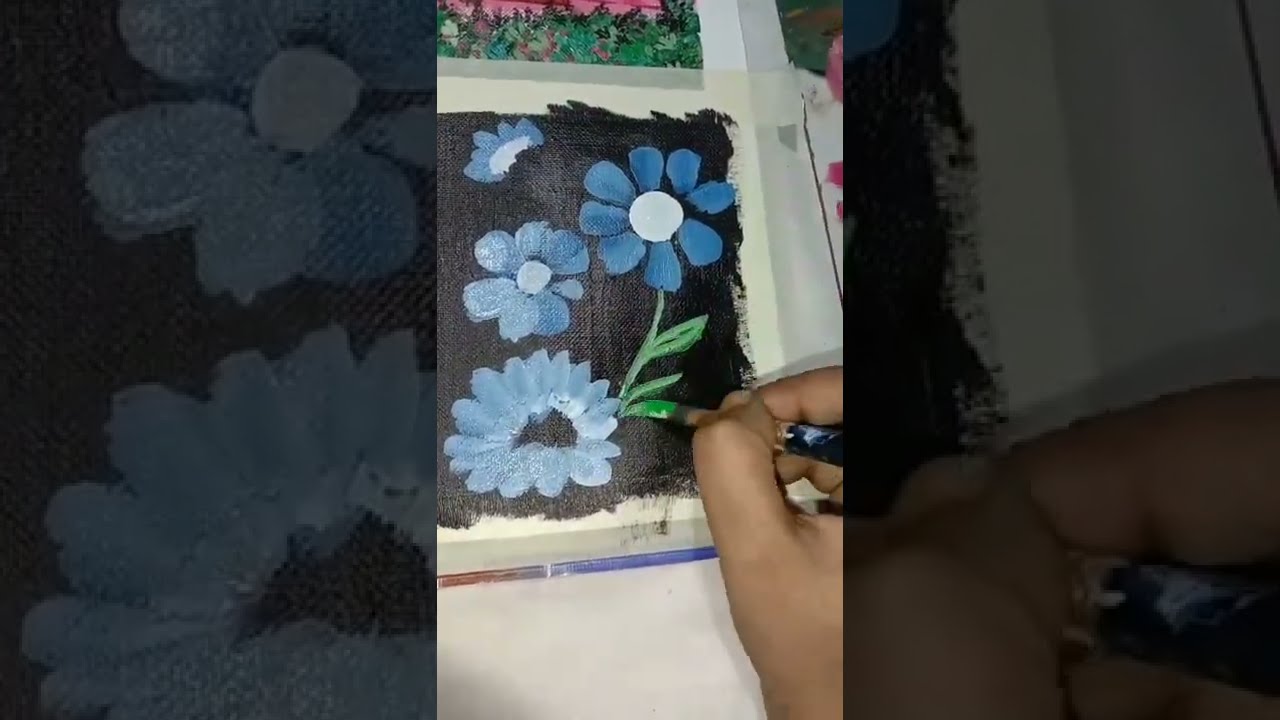The image depicts a person with dark brown skin painting blue flowers on a canvas with a black background. The main focus is a central, vibrant image where the artist's hand, holding a paintbrush with green paint, is in the midst of painting green leaves on the stem of a blue flower. This flower has a white center and eight short blue petals. Around it are partial views of at least three other blue flowers, each differing slightly in their shades of blue and white. Above these flowers, there appears to be what might be the edge of a photograph showing pink flowers, which potentially serves as a reference for the artist. To the right of the central image, there are close-up panels of the painting, darkened for emphasis. These panels showcase blown-up portions of the artwork, highlighting the detailed brushwork and variations in the flower petals. The overall background is white, contrasting the vivid colors and intricate details of the painting.